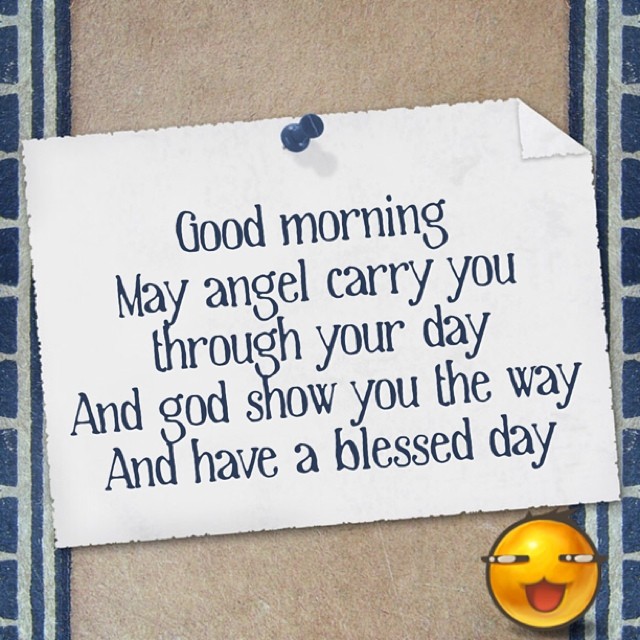The image depicts an illustration mimicking a piece of paper tacked to a textured wall. The central feature is a white piece of paper with rough edges, pinned by a blue thumbtack. The paper bears a caring message in blue text, reading: "Good morning, may angel carry you through your day and God show you the way and have a blessed day," creating a rhyming, uplifting sentiment. In the lower right corner of the paper, there's a cheerful yellow smiley face with an open, orange mouth. The backdrop resembles a bulletin board with a beige central section flanked by vertical blue and white stripes on both sides. The entire composition is square-shaped, contributing to a balanced look that could be recognized as a digital meme or social media sticker designed to inspire positivity.